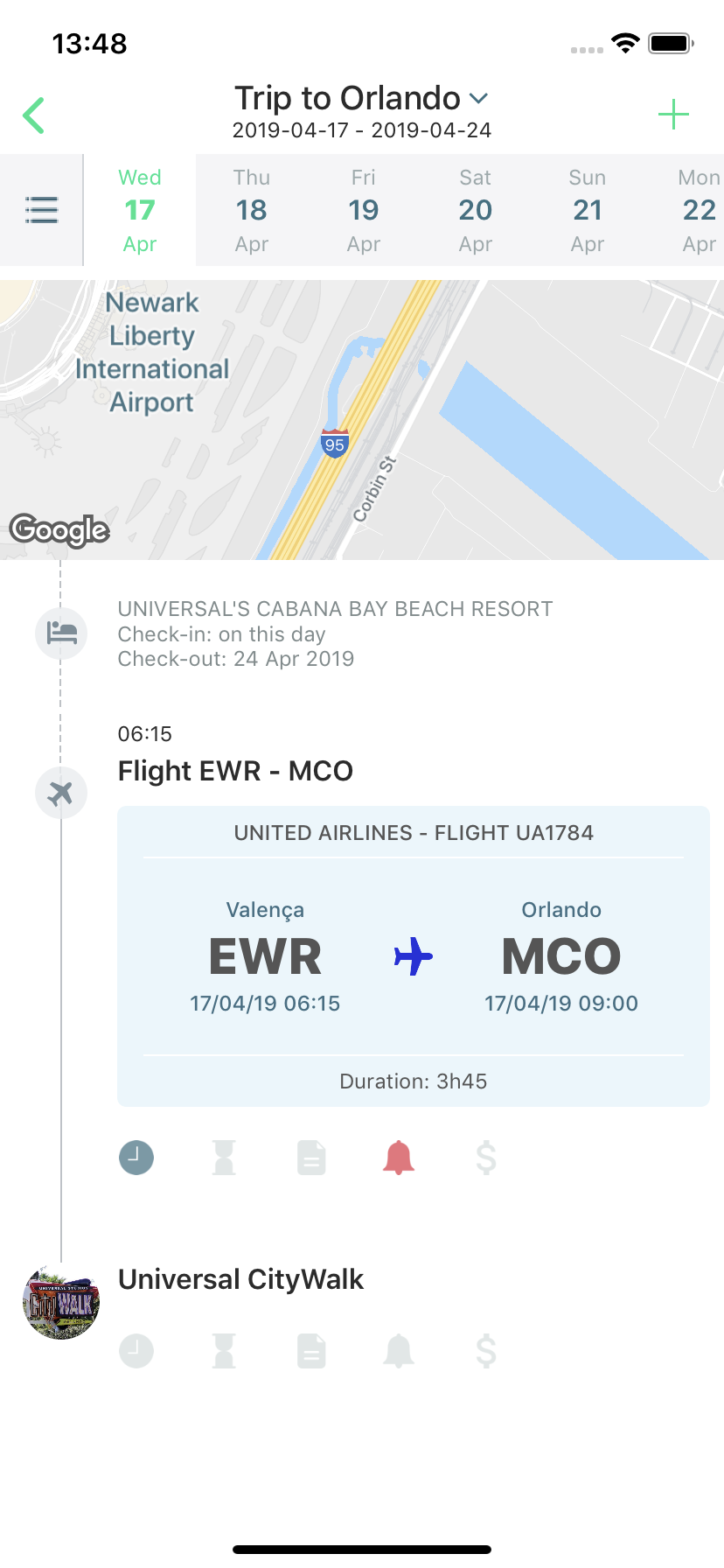### Detailed Caption for the Image

An image displays a smartphone screen showcasing a travel application. At the top, the title "Trip to Orlando" is prominently visible, accompanied by a drop-down menu. The specified travel dates range from April 17, 2019, to April 24, 2019.

On the left side of the screen, there is a green "Back" icon. On the right, a green "+" icon denotes the option to add a new item. Below these icons, a menu icon is situated on the left side. Adjacent to it is a timeline tab with dates displayed in both green and blue, highlighting important trip dates. The date "Wednesday, 17 April" is specifically marked in green, while the subsequent dates from "Thursday, 18 April" to "Monday, 22 April" are highlighted in blue.

Directly below this section, a detailed map is displayed. On the left part of the map, it states "Newark Liberty International Airport," followed by some text which might indicate altitude or a related metric. Underneath the map, the text indicates lodging details at "Universal Cabana Bay Beach Resort," with a check-in date of April 17, 2019, and a check-out date of April 24, 2019.

The itinerary details are listed below this information:
- **Flight Itinerary:**
  - **Departure:** April 17, 2019, at 06:15 AM from Newark Liberty International Airport (EWR).
  - **Airline:** United Airlines, Flight Number UA-1784.
  - **Arrival:** April 17, 2019, at 9:00 AM at Orlando International Airport (MCO).
  - **Flight Duration:** 3 hours 25 minutes.

In the middle of the screen, the flight information is further emphasized in a blue highlight, providing clarity on departure, arrival, and flight duration. 

At the bottom edge of the application screen, there are icons for different functionalities such as "Time," "Notification," and "Price." The final segment on the screen features the text "Universal CityWalk," indicating a notable destination or event on the travel itinerary. This travel application appears to be tailored for efficiently organizing and managing trip details.